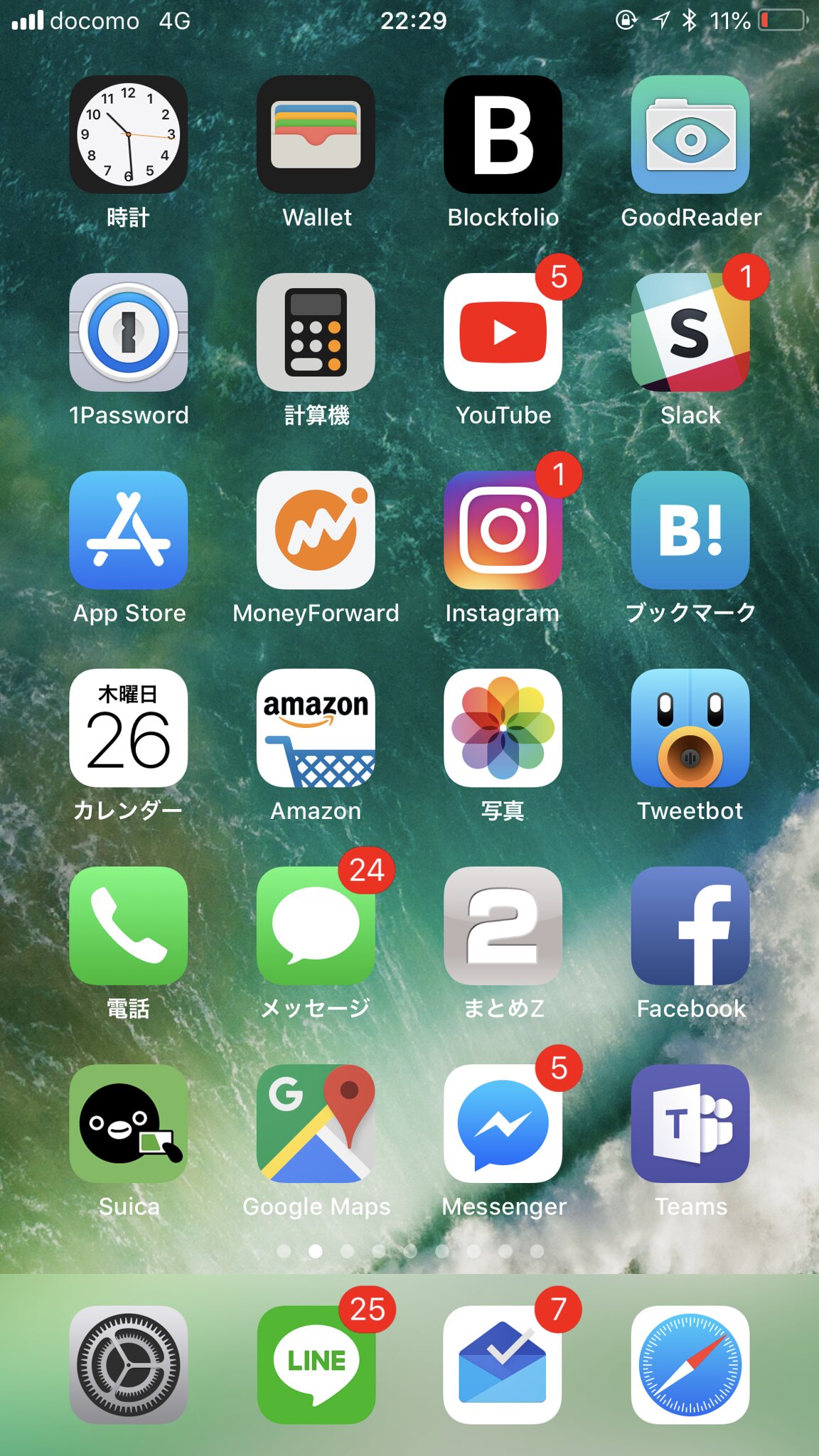Screenshot of a smartphone home screen featuring a diverse array of apps. The display is organized into seven rows of apps against a bluish-green background with white highlights, likely depicting an ocean scene. At the top of the screen, network indicators show a strong Wi-Fi signal, the carrier name "DOCOMO," and a 4G connection. The clock displays 22:29. A series of icons, including a navigation icon and several small symbols, appear on the right alongside a critically low battery level at 11%, indicated by a red bar.

The apps are a mix of English and East Asian script, suggesting possible Chinese or Japanese origins. The English-labeled apps include: wallet, Blockfolio, GoodReader, 1Password, YouTube, Slack, App Store, Money Forward, Instagram, Amazon, Tweetbot, Facebook, Suisa, Google Maps, Messenger, and Teams. The app icons are vibrantly colored, including blues, greens, yellows, blacks, reds, oranges, and purples. Many apps display red notification bubbles, indicating pending alerts or messages.